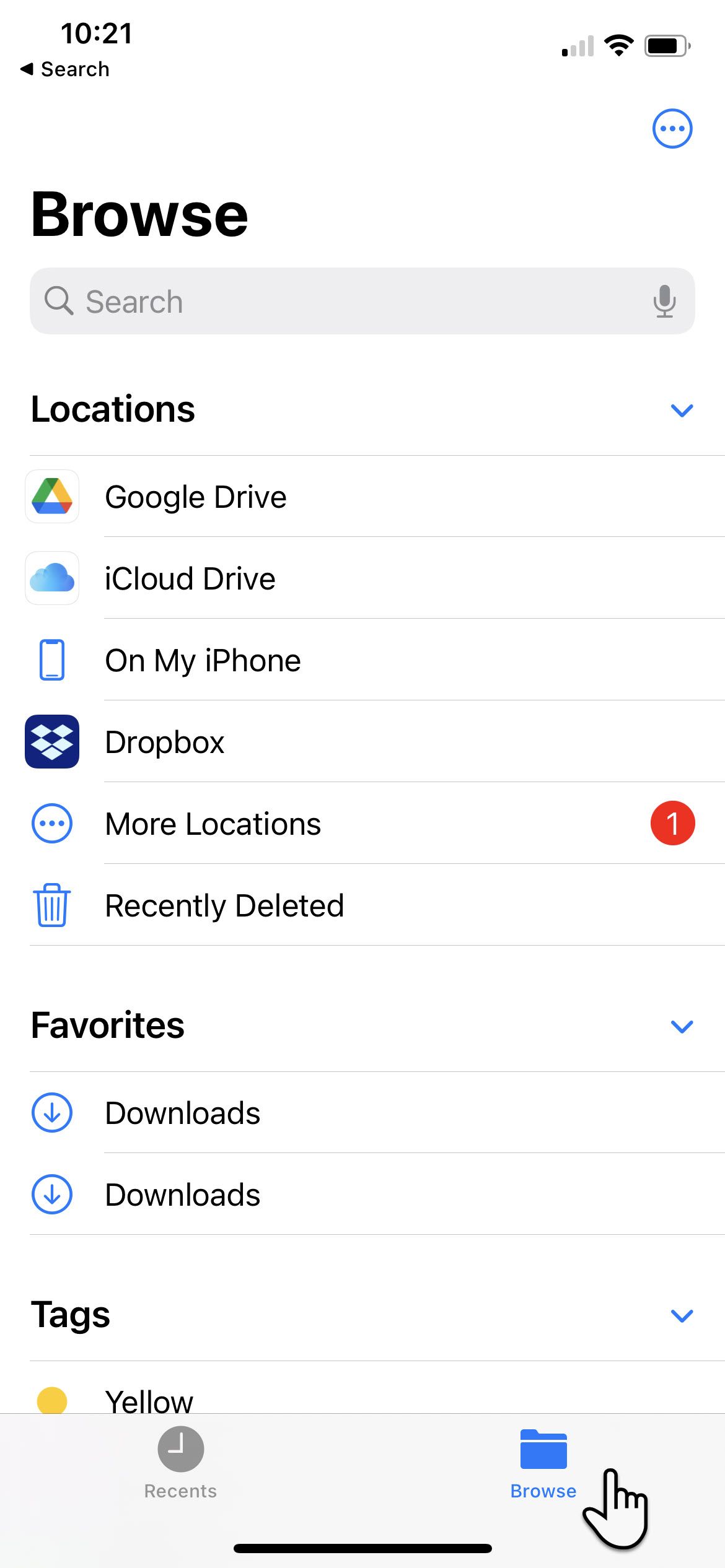The image showcases a screenshot of a mobile device interface. At the top left corner, the time displayed is 10:21. On the top right, the icons indicate network signal strength, WiFi connection, and the current battery level. The main section of the screen features a file management app with several navigational options. These options include "Browse," "Locations," "Google Drive," "iCloud Drive," "On My Phone," "Dropbox," "On Locations," "Recently Deleted," "Favorites," "Downloads," "Recents," and again "Browse." A cursor is actively positioned on the "Browse" button, indicating user interaction.